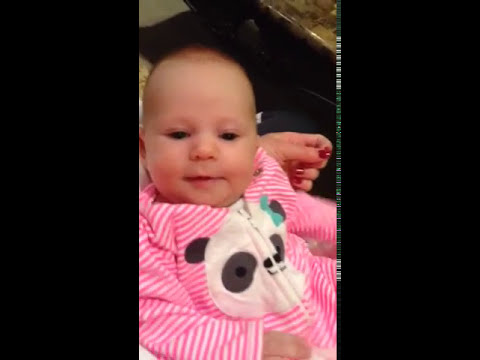The image captures a close-up of a young baby, likely a few months old, with short, reddish hair and chubby cheeks. The baby is wearing a pink and white striped onesie with a zipper down the middle, adorned with a smiling panda bear that has gray eyes, gray ears, a black nose and mouth, and a small green or blue ribbon on its head. The baby's right hand is visible, slightly extended from the sleeve. 

To the right of the baby's left shoulder, there is an adult hand, likely a woman’s, with red fingernail polish, suggesting the baby might be resting on the woman's chest. The baby appears relaxed and is facing towards the camera, not directly staring but looking slightly downward. 

The photo shows the baby centered within a wide rectangular frame, framed on either side by wide black vertical bands. The background includes a shiny brown countertop or desk, adding context to the cozy, indoor setting.